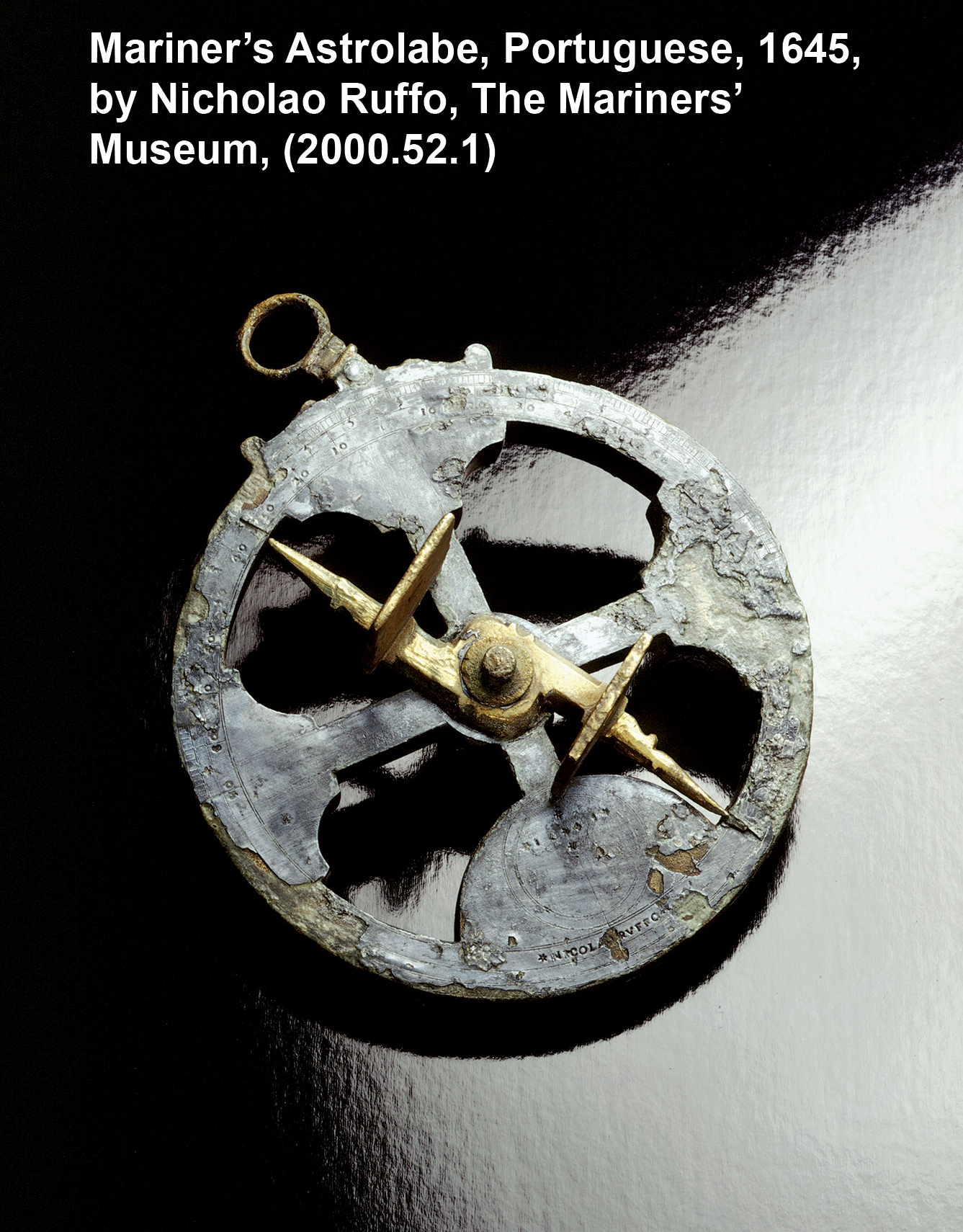This detailed image captures an ancient navigational tool called a Mariner's Astrolabe, attributed to Nicolao Ruffo in 1645, and held by The Mariner's Museum (catalog number 2000.52.1). The astrolabe, made of metal with a gold center, is noticeably worn and weathered, suggesting its extensive historical use. It is round and features a loop at the top, likely for attaching a strap. The front surface is etched with intricate, map-like engravings and arrows, which hint at its function in maritime navigation. The background is split with the left side and parts of the right being black, while the center-right portion is gray. The identifying text is presented in white over the black sections, creating a stark contrast that emphasizes the age and provenance of this fascinating artifact.